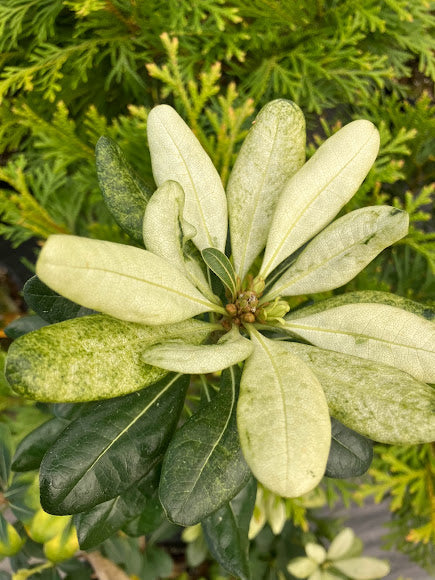This close-up photograph captures a vibrant and detailed view of a pittosporum plant, specifically highlighting its variegated leaf pattern and subtle floral elements. The plant in the foreground features an array of leaves that transition from very light, almost white, green to a darker green beneath. These variegated leaves showcase a speckled pattern with darker green accents and have a striking contrast with the under layer, which is a flat, dark green. In the center of the plant, small olive and dark brown blossoms are beginning to bloom, with some showing a subtle gradient from dark brown to light brown as they fade into the surrounding green foliage.

The backdrop of the image includes various trees, possibly a cypress or similar evergreen, providing a lush, green contrast to the lighter leaves of the foreground plant. Notably, smaller branches that appear furry and small branches coming off of these are visible, contributing to the intricate texture. There's also a hint of the garden's earthy ground, signifying the natural setting.

The overall scene is bathed in bright sunlight, enhancing the vivid greens and ensuring that the primary subject remains in sharp focus while the background features a gentle lens blur, emphasizing the rich details of the pittosporum. The interplay of sunlight and shadow denotes a daytime capture, further enriching the image's brightness and contrast.